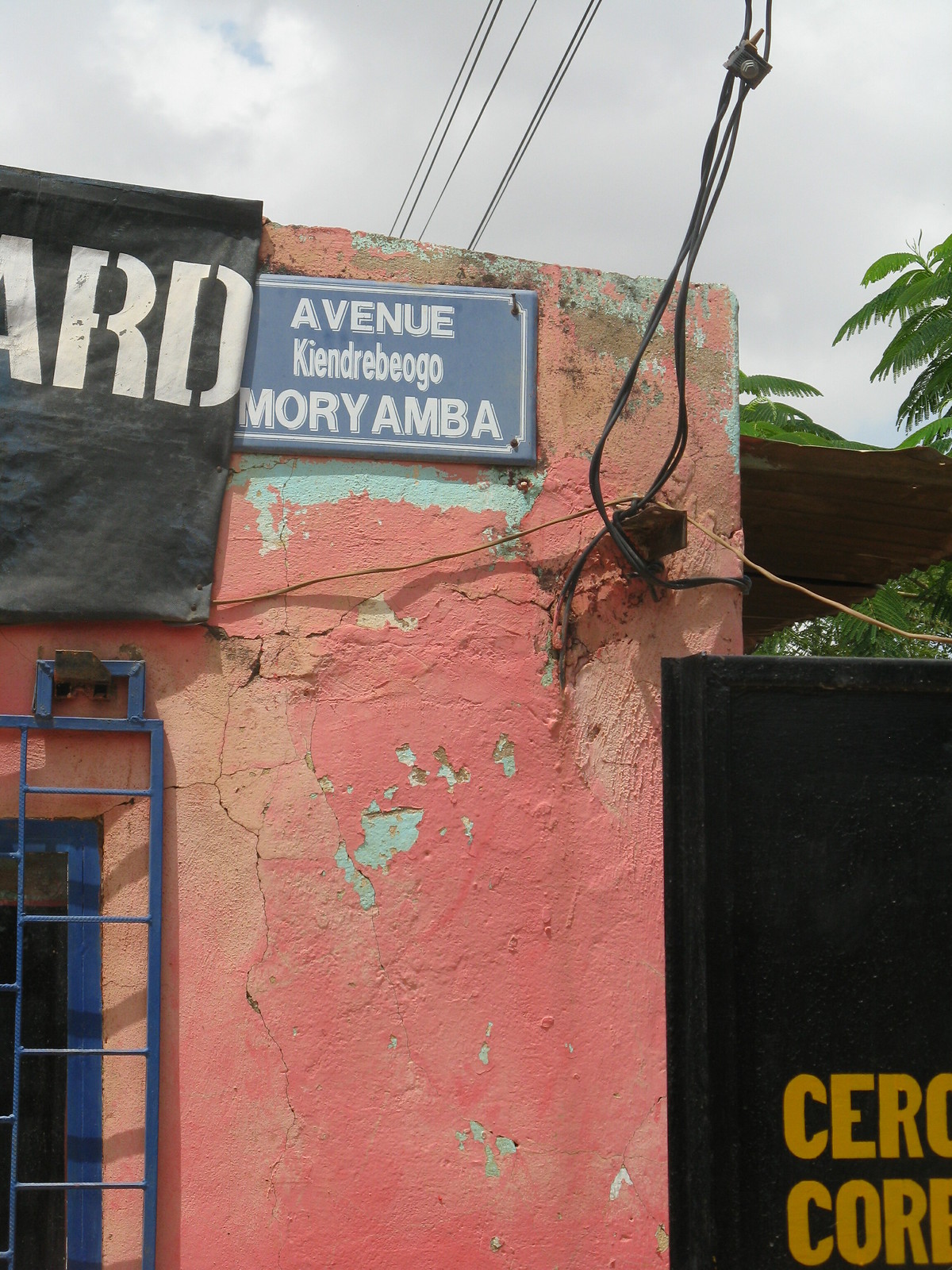This outdoor image captures the corner of a weathered, stone building. The building's faded salmon-colored paint is chipped, revealing patches of an older turquoise layer beneath. The walls are visibly cracked, enhancing the structure's rundown appearance. Dominating the lower left section of the image, a window framed with blue bars stands out, though it’s partially obscured. Power lines extend from the building’s corner, intersecting the scene with stark black lines. Affixed to the side of the building is a blue sign with white lettering that reads "Avenue KENDRE BEOGO MORIYAMBA," although a few characters are slightly misaligned, making the exact spelling somewhat ambiguous. Adjacent to this, a black billboard prominently displays the letters "A-R-D" in white.

In the bottom right corner, another black sign is visible, this one with cut-off yellow letters reading "C-E-R" and "C-O-R-E." The sky above is a bright blue, dappled with fluffy white clouds. To the right side of the image, lush, green tropical trees blend into the scene, adding a touch of nature to the urban environment. An awning matching the building’s pinkish hue also peeks into view from the right. This intricate mix of details creates a vivid portrayal of a possibly commercial structure, hinting at a store or possibly a pawn shop, shaped by time and elements.